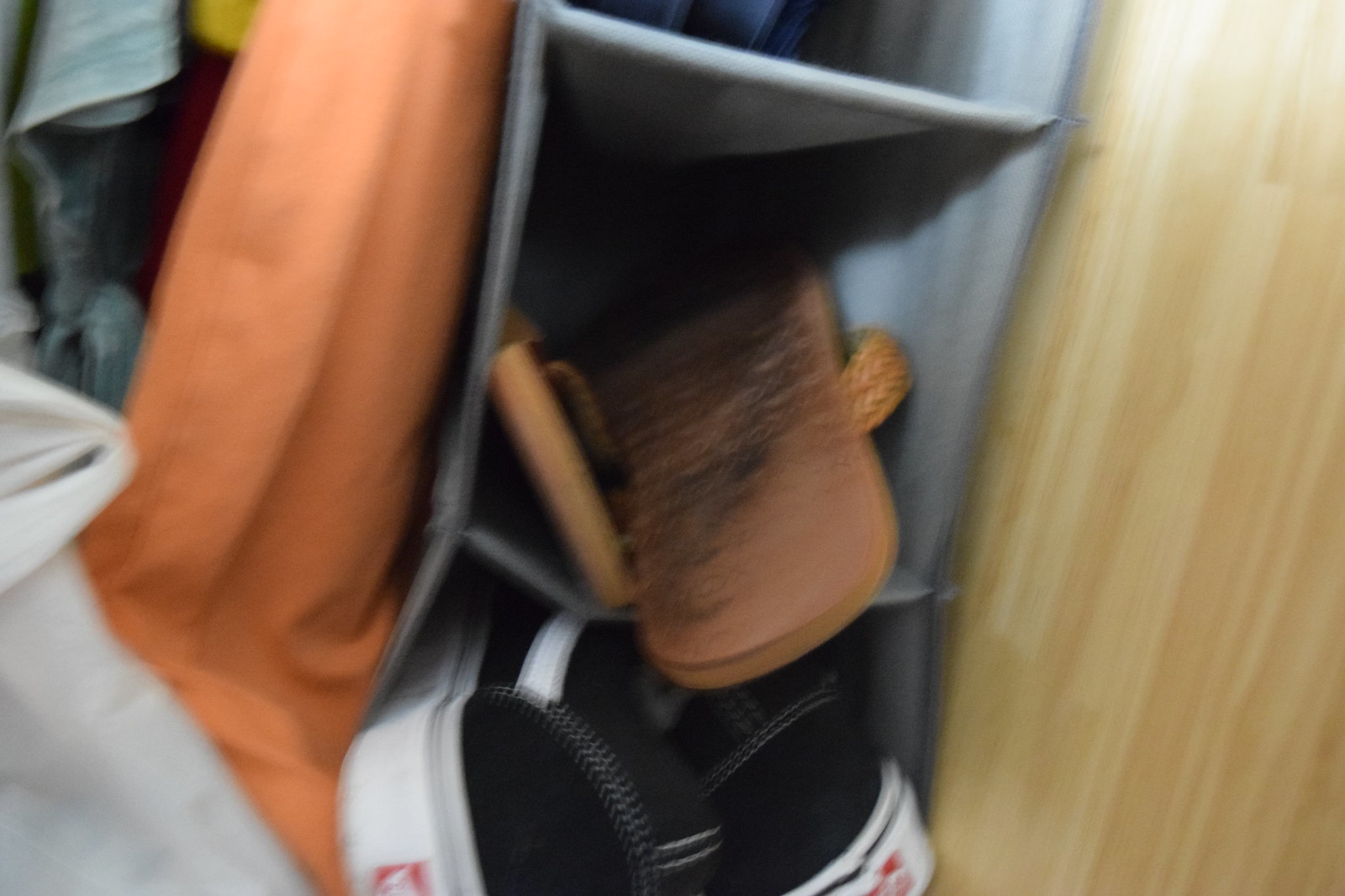This blurry photograph captures an inside view of a closet, likely taken with the camera held at an angle. On the right side, a vertical light blonde wood panel is visible, possibly part of a door or wall. Central to the image is a gray fabric shoe cubby, hanging from an overhead clothes bar. Three of the cubbies are visible: the top one shows the tip of dark-colored shoes, the middle cubby contains a pair of brown sandals with noticeably dirty, blackened soles, and the bottom cubby holds a pair of black sneakers with white trim and soles, featuring a fuzzy red logo on the heel. To the left of the shoe cubby, an orange piece of fabric hangs, and partial shirt sleeves are visible in the upper-left corner. The lower-left corner shows a patch of white, possibly another garment or fabric item.